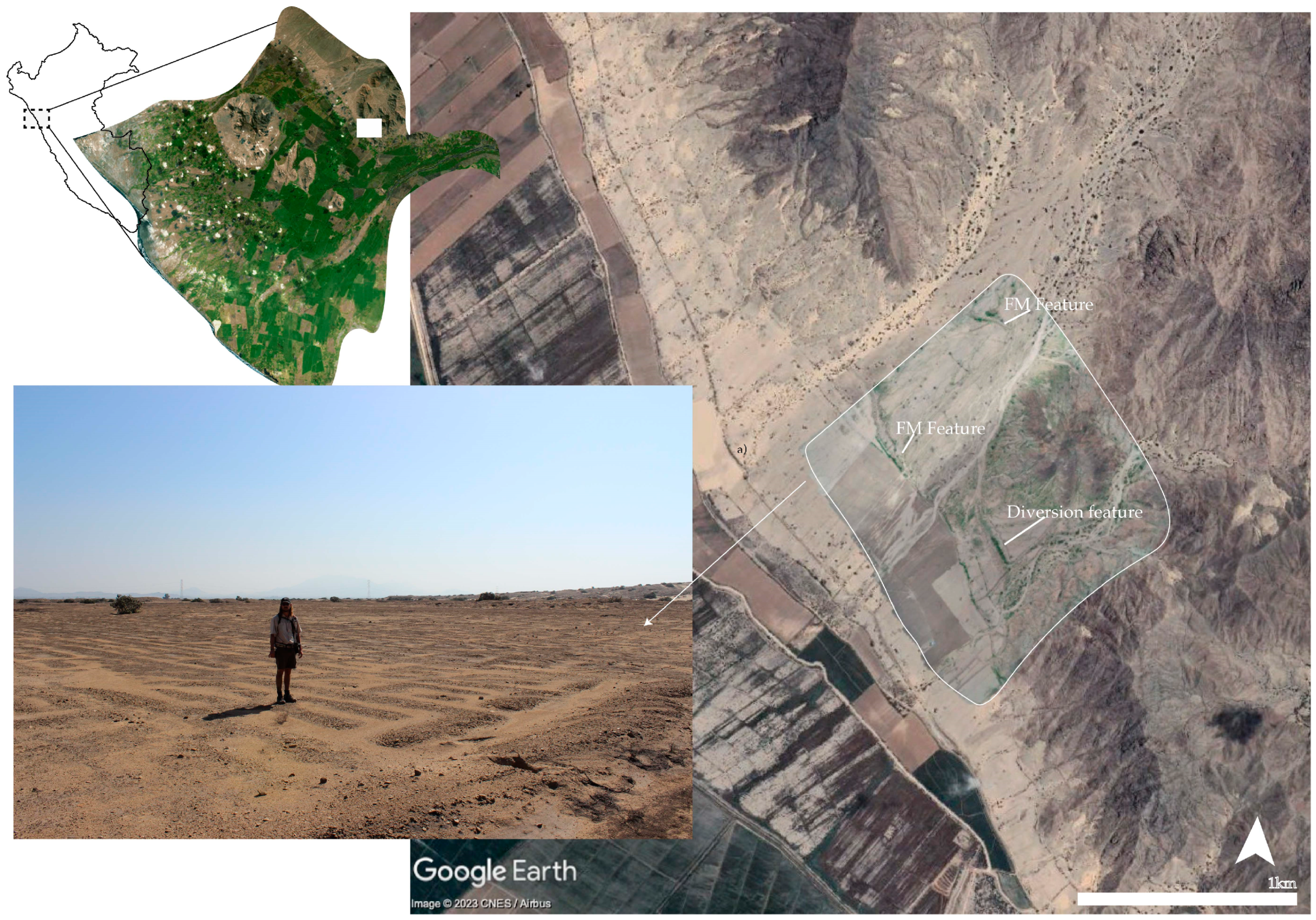The image is a composite of aerial and ground-level perspectives, primarily showcasing a Google Earth view of rugged terrain. The main body of the picture is a top-down view of a desert-like landscape with varying shades of browns, tans, blacks, and rusty colors, highlighted by lines and a light green diamond shape, indicating specific features labeled as "FM feature" and "diversion feature." These features are partially illegible. An inset to the left reveals an upside-down diamond-shaped diagram with green land and a white strip, linked by lines and a small box. Below this, a rectangular photograph juxtaposes a lone person standing on the landmass against a clear blue sky without clouds, an arrow pointing down confirming their location. Additionally, a small legend at the bottom indicates a scale of one kilometer with an upward arrow. Overall, the image weaves together detailed geographical and human elements within a desolate yet visually complex landscape.